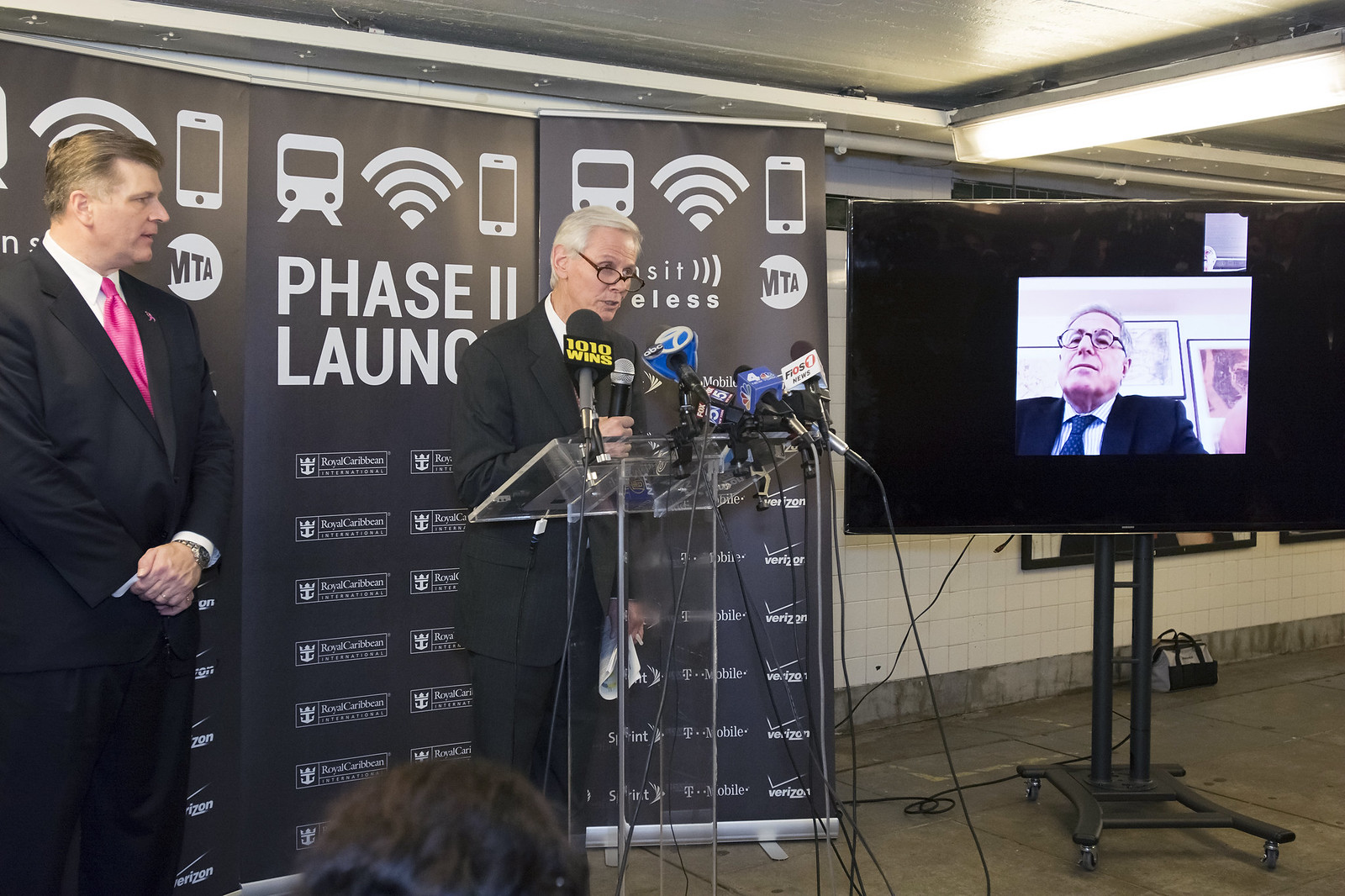The image depicts an indoor setting, likely a press conference or official announcement. On the left side, an elderly Caucasian man with white hair, black glasses, and a blue tie stands behind a plexiglass podium crowded with around seven microphones from various news stations. He is in a black suit and white dress shirt, addressing an audience, with a banner behind him that reads "Phase II Launch." The banner also features symbols for a transit bus, Wi-Fi signal, cellular bars, and a phone, suggesting a technology or transportation announcement.

To his left, another man stands, slightly taller and heavier set, with light brown hair graying at the temples. This man, also in a black suit with a white dress shirt, has a red tie and his hands crossed over his lower stomach, looking towards the speaker.

On the right half of the image, there is a black television monitor mounted on a metal podium with wheels. The monitor shows a video call featuring an older man wearing a suit and tie. Additionally, a smaller image of another participant is visible in the top right corner of the monitor. The overall scene suggests a multi-participant announcement involving both in-person speeches and remote communication, likely regarding a significant technological initiative or company milestone.